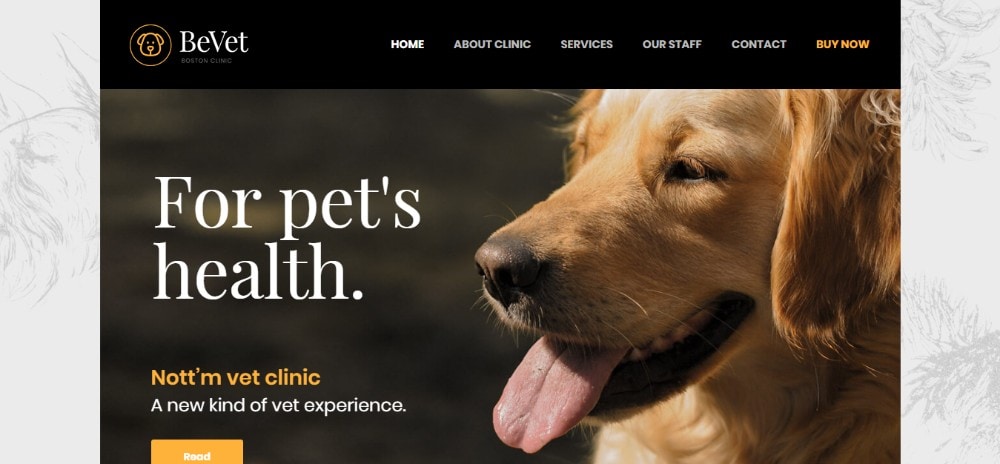This screenshot captures the polished landing page of BeVets, a veterinary company. Dominating the header, an elegant black bar spans the top, prominently featuring the BeVets logo—a simplistic yet striking outline of a dog's face in orange—situated on the far left. Adjacent to the logo, a streamlined menu bar offers easy navigation with options labeled: Home, About Clinic, Services, Our Start, and Contact. On the far right, a standout "Buy Now" button in vivid orange grabs attention.

The page's background is adorned with a heartwarming image of a golden retriever, its playful tongue lolling out, positioned on the right side of the screen. To its left, a set of compelling white text reads, "For Pets' Health," followed by a smaller, eye-catching orange line that says, "Not Now, Vet Clinic." Just beneath that, a tagline in white, "A new kind of vet experience," appears, encapsulating the clinic's innovative approach. This section of text is punctuated by an inviting orange "Read More" button. Overall, the design melds a clean, professional aesthetic with a touch of warmth, perfectly reflecting the brand’s mission.